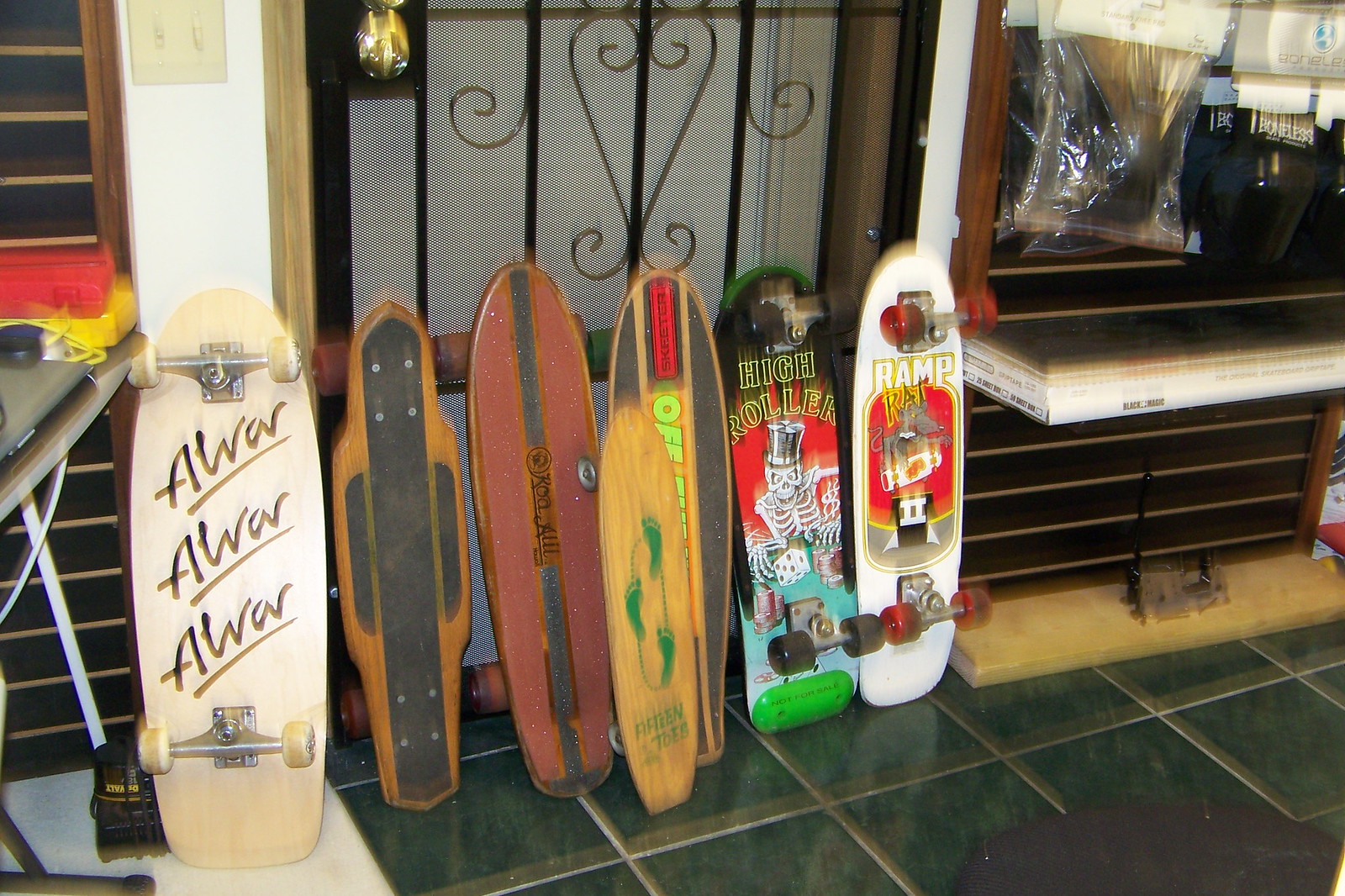This photograph captures a variety of skateboards propped up against a black metal grated door with a heavy-duty doorknob. The ground features black tiles, adding contrast to the vibrant lineup of boards. From left to right, you'll notice a wide, round skateboard with a wooden texture that has the phrase "A WAR A WAR A WAR" underlined in black and white text. Adjacent to it is a narrow, angular skateboard followed by a striking red board with a green stripe. A tiny wooden board with green bindings is next, and another board prominently displays "HIGH ROLLER" beneath an image of a skeleton wearing a top hat. Accompanying these is a board branded "RAMP RAT," showcasing a rat riding a skateboard against a red background with red wheels. The arrangement includes a variety of other longboards and a makeshift penny board, reminiscent of the types used along Venice Beach or L.A. Boulevard. On the right side of the image, some accessories including a plastic bag and knee pads are visible on a rack. Despite the shakiness of the photo, the eclectic mix of skateboard shapes, colors, and designs is evident, showcasing everything from classic grip tape and bolts to unique graphics and vibrant decks.